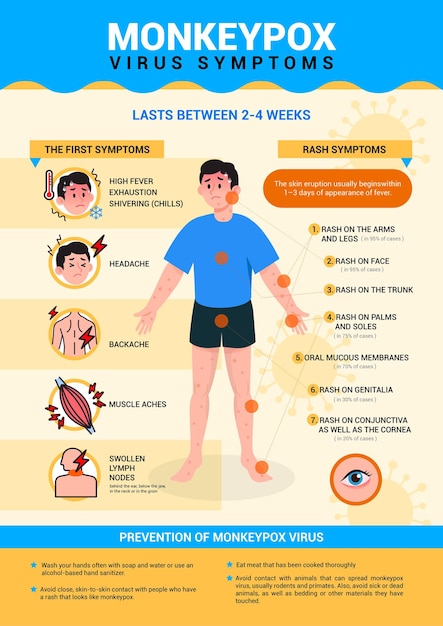The digital poster, headered with "Monkeypox Virus Symptoms" in white on a sky blue background, details critical information through a colorful and structured design. The poster is divided into several sections with distinct color schemes. Below the header, the text states the illness "lasts between 2 to 4 weeks" on a wavy off-white background with a hint of yellow at the waves' edges. An orange ribbon labeled "The First Symptoms" introduces a section listing early signs, including high fever, exhaustion, shivering, chills, headache, backache, muscle aches, and swollen lymph nodes, each represented by icons of affected body parts.

On the right side, under the title "Rash Symptoms," details of the rash progression are provided, illustrated by an orange blob. A central figure of a man in a blue shirt and black shorts is marked with numbered labels pointing to rash locations: arms, legs, face, trunk, palms, soles, oral mucus membranes, genitalia, conjunctiva, and cornea. 

The lower section of the poster, starting with a blue horizontal strip, covers "Prevention of Monkeypox Virus" in white text. Further details in an orange section with blue stars advise on preventive measures: frequent hand washing with soap and water or using alcohol-based sanitizers, avoiding close skin-to-skin contact with those showing a rash, thoroughly cooking meat, and avoiding contact with rodents, primates, sick or dead animals, and their bedding. The poster combines visual aids and text in sky blue, white, black, yellow, and orange to provide a comprehensive guide on the symptoms and prevention of monkeypox.